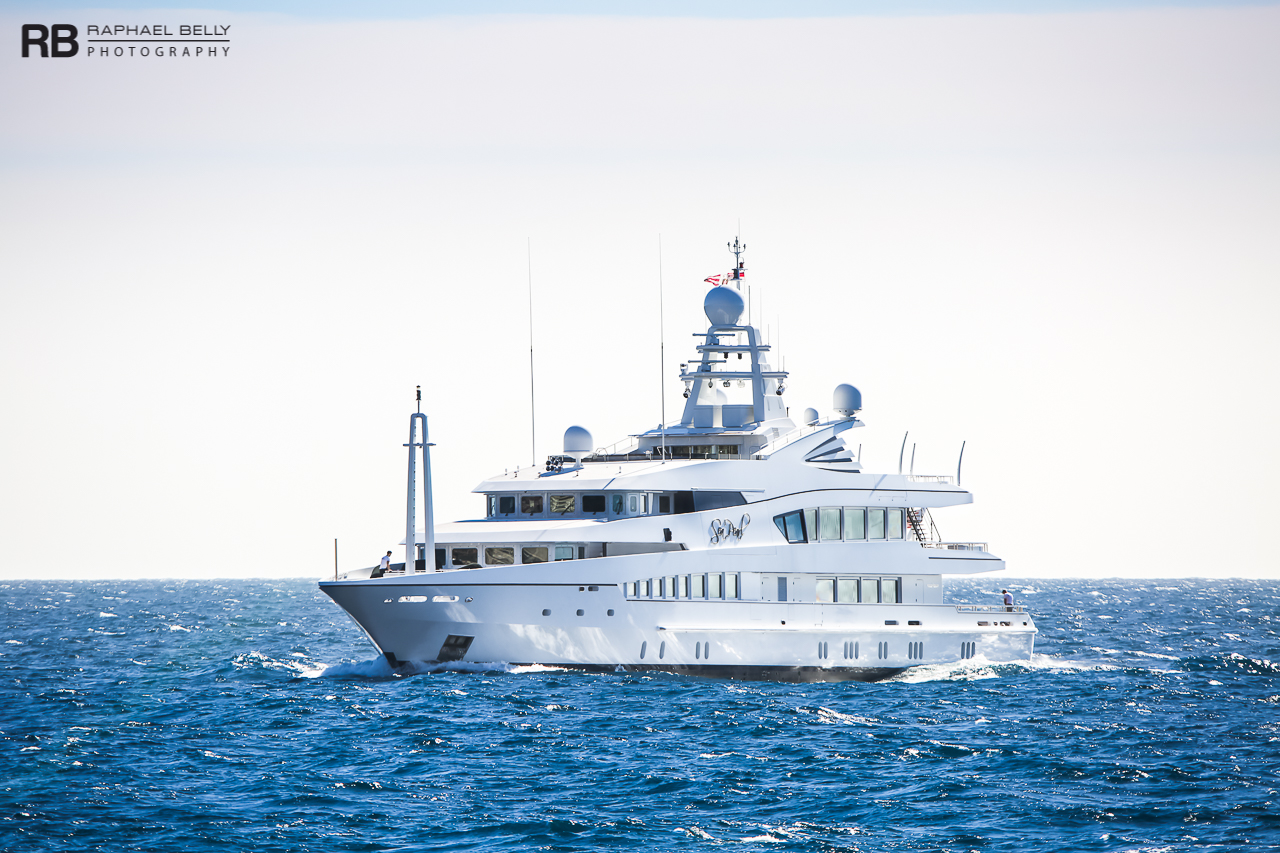The image depicts a luxurious and sleek power boat cruising through the sea on a beautifully sunny day. The waters, stirred by the wind, exhibit some waves, adding a dynamic element to the scene. The boat itself is exceedingly large and modern, characterized by its rounded front and extensive array of windows spanning both levels of the vessel. 

On the bow of the deck, a person is seen walking back towards the ship, while another individual occupies the back deck. Atop the boat, an impressive collection of radar and sonar equipment is visible, signifying the advanced technological capabilities of this vessel. The flybridge, offering elevated sightlines, indicates a space where someone can enjoy panoramic views of the surroundings. 

A distinctive U-shaped design element is present on the front of the boat, complemented by a prominent light fixture that extends above the vessel. Additionally, the ship is flying several foreign flags, further enhancing its sophisticated and contemporary appearance. The overall ambiance of the image suggests a perfect day for sailing aboard this state-of-the-art, brand new boat.